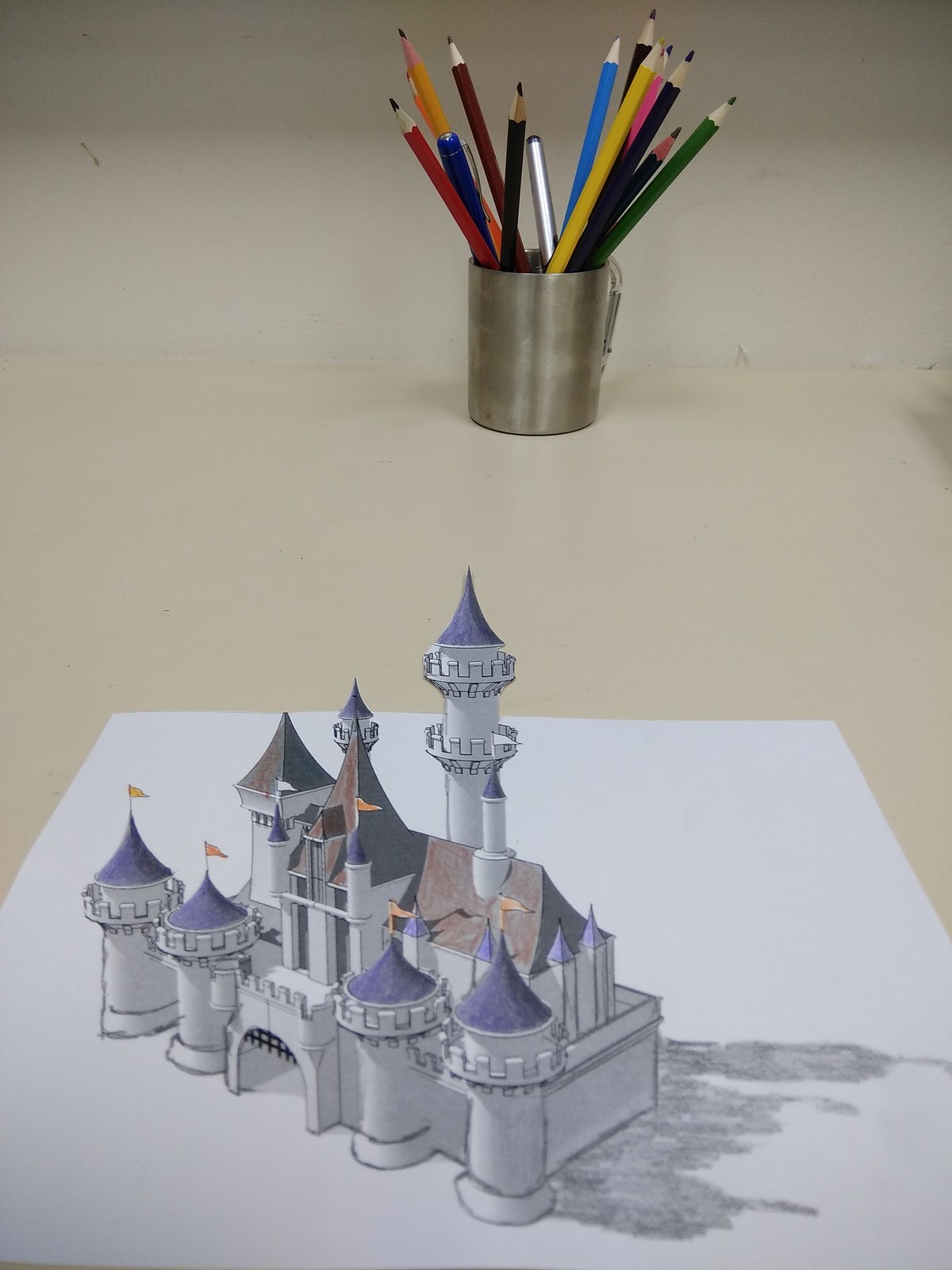The image shows a detailed sketch on a white piece of paper, placed on an off-white colored table. In the background, there is a slightly tarnished, silver metallic cup holding a variety of colored pencils with their pointed ends upwards. The cup contains pencils in several colors including blue, yellow, green, brown, black, pink, and some regular pencils, along with an ink pen and a blue marker. The centerpiece of the drawing is a grayish castle with a 3D effect, enhanced by its tallest tower extending off the paper. The castle features four front towers with blue roofs and small yellow-orange flags. The central gate of the castle is open, inviting viewers into its detailed structure. There is a shadow cast towards the right, contributing to the realistic look, while the tallest tower in the back, presumably purple based on descriptions, adds depth to the piece. The background of the image also includes a faintly visible light beige wall, enhancing the overall composition.